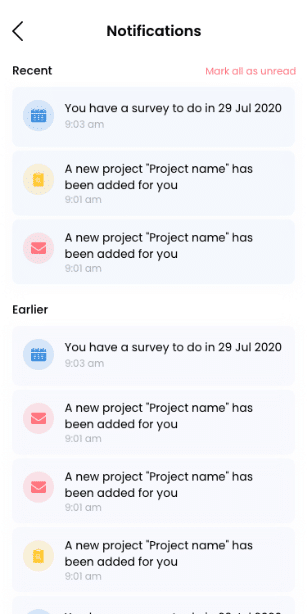The image appears to be a screenshot of a smartphone notification page. At the top of the screen, there is a left-pointing arrow. Next to the arrow, the word "Notifications" is displayed in black font. 

Below this, "Recent" is written in black font, accompanied by a red text option that reads "Mark all as unread." 

The notifications are listed with various icons and messages:
1. An icon of a blue calendar is followed by a message, "You have a survey to do on 29 July 2020 at 9:03 a.m."
2. An icon of a yellow shopping bag includes the message, "A new project 'Project Name' has been added for you at 9:01 a.m."
3. A red mail envelope icon states, "A new project 'Project Name' has been added for you at 9:01 a.m."
4. Repeated notifications follow with the same text and differing icons:
   - Blue calendar: "You have a survey to do on 29 July 2020."
   - Red mail envelope: "A new project 'Project Name' has been added for you at 9:01 a.m."
   - Red mail envelope: "A new project 'Project Name' has been added for you at 9:01 a.m."
   - Yellow shopping bag: "A new project 'Project Name' has been added for you at 9:01 a.m."